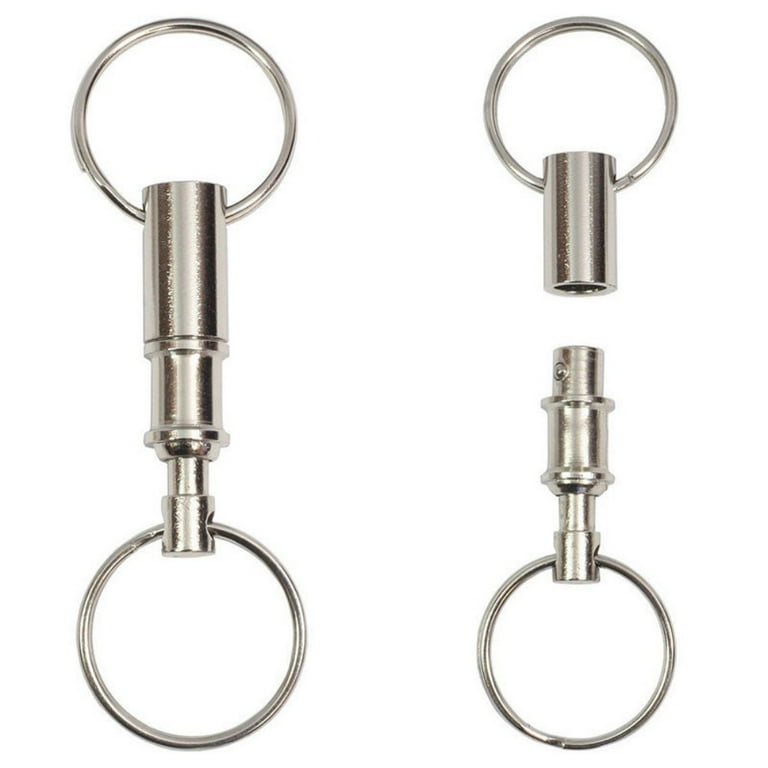This image features a pair of detachable keychains, each consisting of a silver-colored cylindrical barrel with rings on both ends. The keychain on the left is shown fully assembled and positioned vertically, showcasing its sleek, metallic design. The top and bottom rings are securely connected by the barrel in between. In contrast, the keychain on the right is separated into two parts, revealing the internal mechanism. This mechanism includes a small ball that locks into place when the pieces are connected, demonstrating how the assembly and disassembly function. The shiny chrome finishes of both keychains contrast sharply against the bright, white background.